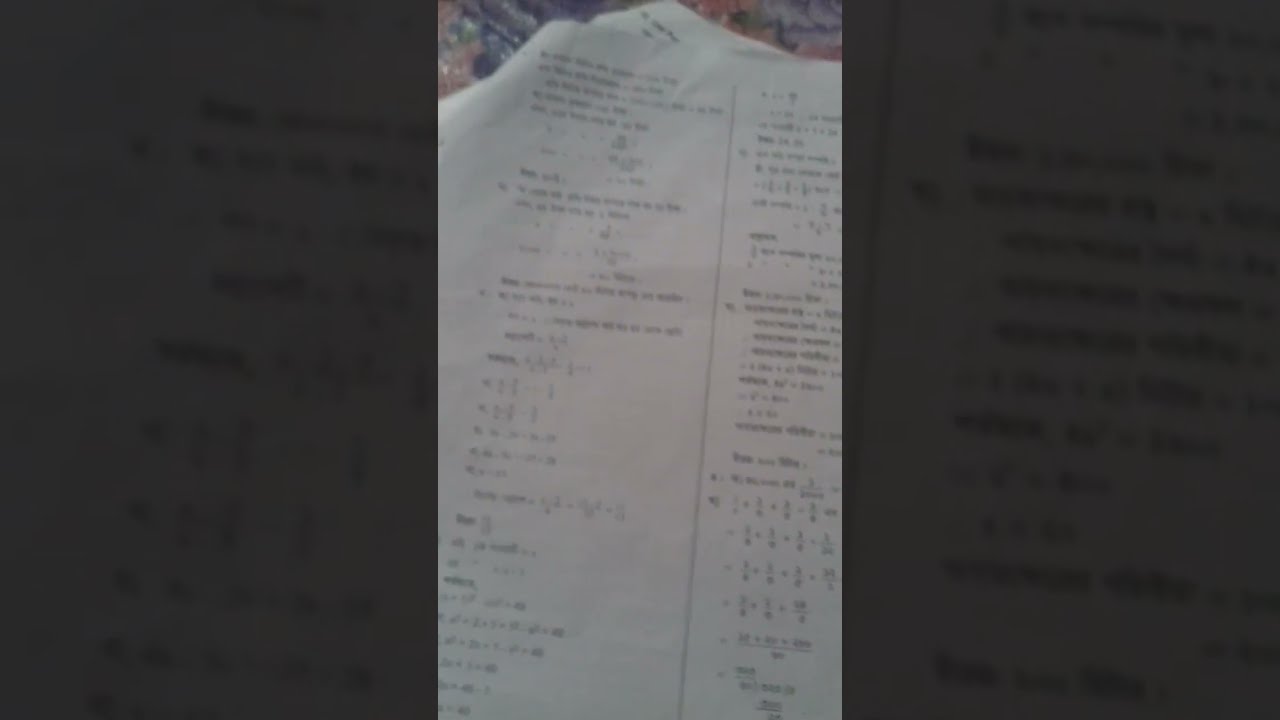The image consists of two photos of the same scene, with one serving as a darker, zoomed-in background of the primary photo in the middle. The central image is formatted vertically to fit the size of a phone screen, displaying a folded worksheet, likely a schoolwork page. This page appears to be math homework focused on multiplying fractions, with problems numbered and answers labeled A, B, C, D, and E. The white sheet features black text, which is arranged in two columns and slightly blurred, making specifics hard to discern. A line runs down the middle of the page, enhancing the division of columns. The sides of the main image are gray and blurred, while the bright background includes shades of crystal blue and pink at the top. Some discernible fractions and numbers include "2 over 6," "3," and potential sums like "2 over 8 plus 3 over 9." The overall context suggests a classroom or home study environment.